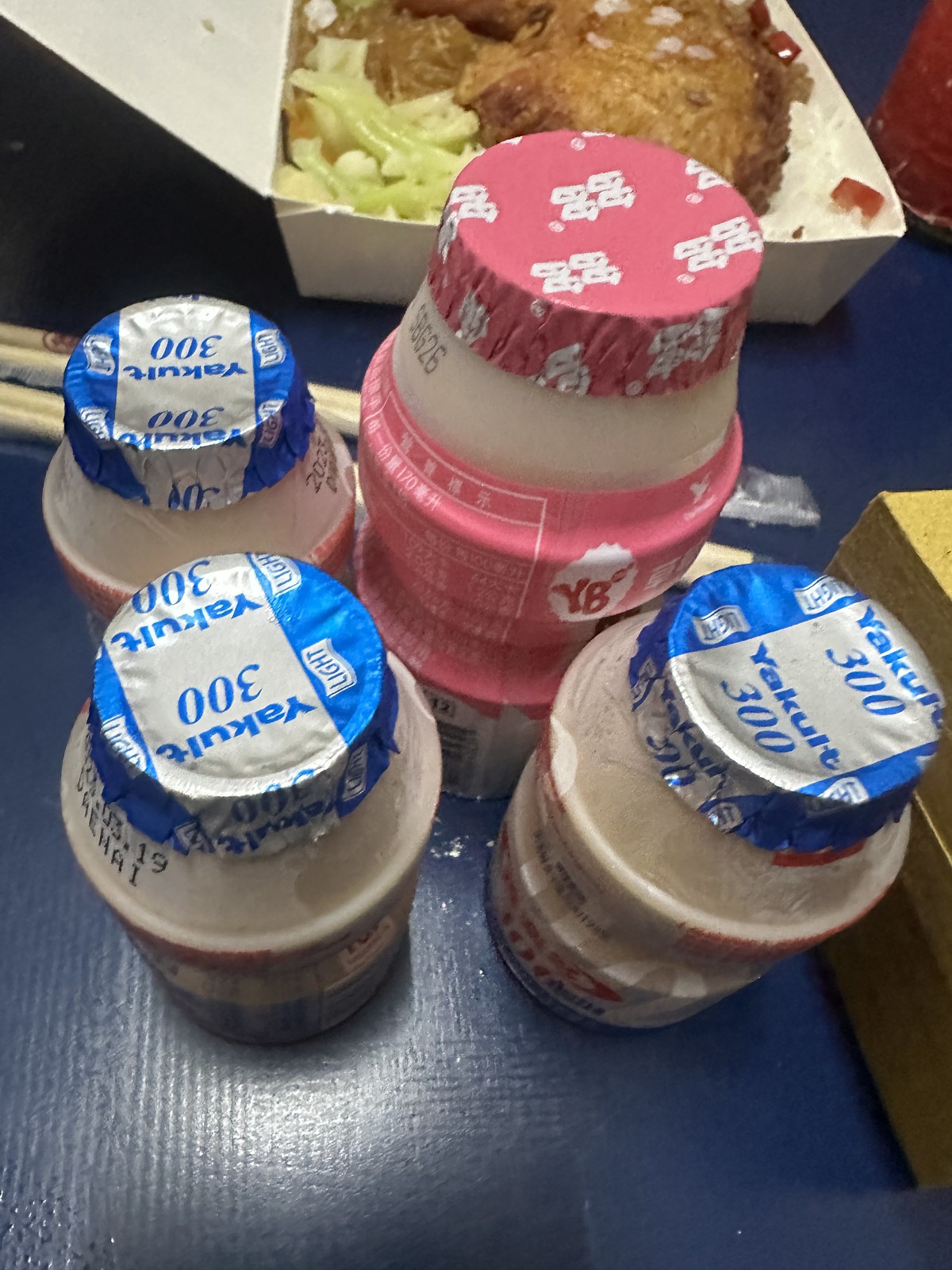This color photograph, taken with a personal camera, features a set of four beverage bottles prominently displayed on a blue surface. The central bottle is taller and wrapped in a pink foil, indicating it might be strawberry-flavored milk or yogurt. It displays a capital "Y" and "B" on its white background. Surrounding it are three smaller bottles, each with a white body and a blue and silver peel-off foil lid, bearing the words "Yakult 300" and "Light" in metallic blue text. These bottles are likely yogurt drinks.

Behind these bottles, there are two pairs of unused chopsticks and a white takeout container partially filled with what seems to be an assortment of fried food, rice, and possibly some chicken or noodles. The takeout box spans the top center of the image and extends about a third of the way down, revealing items like a greenish-yellow vegetable on one side and a white food item on the other. The background also includes other colorful elements, such as a red item in the upper right corner and a yellow block in the lower right.